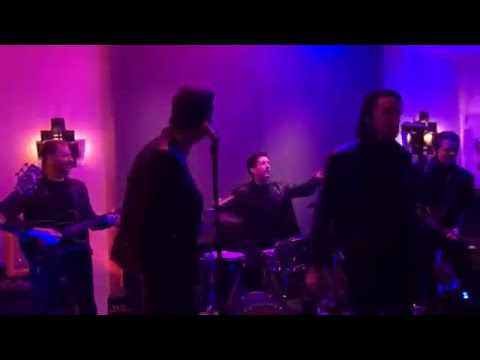The image captures a musical band performing on a dimly lit stage, likely in a bar or club. The setting is suffused with a moody ambiance created by gradient lighting in hues of pink, purple, and blue. The image quality is somewhat low, appearing grainy and small, suggestive of a still from a low-resolution video. The band consists of five men, all dressed in black attire, predominantly leather jackets.

Central to the image is the drummer, actively playing and positioned at the heart of the performance. To his left, a guitarist strums away, while to the drummer's right, another musician appears to be playing a keyboard, also seated. Two men, each standing in front of a tall microphone, dominate the forefront of the image. One of them is turned towards the drummer, possibly engaging with the beat, while the other faces forward, likely singing. A bass player is visible at the left edge of the frame, partially obscured but discernible by his position and instrument. The smoky atmosphere, coupled with violet and purple spotlights at the back, envelops the scene, enhancing the band's compelling and intimate performance.